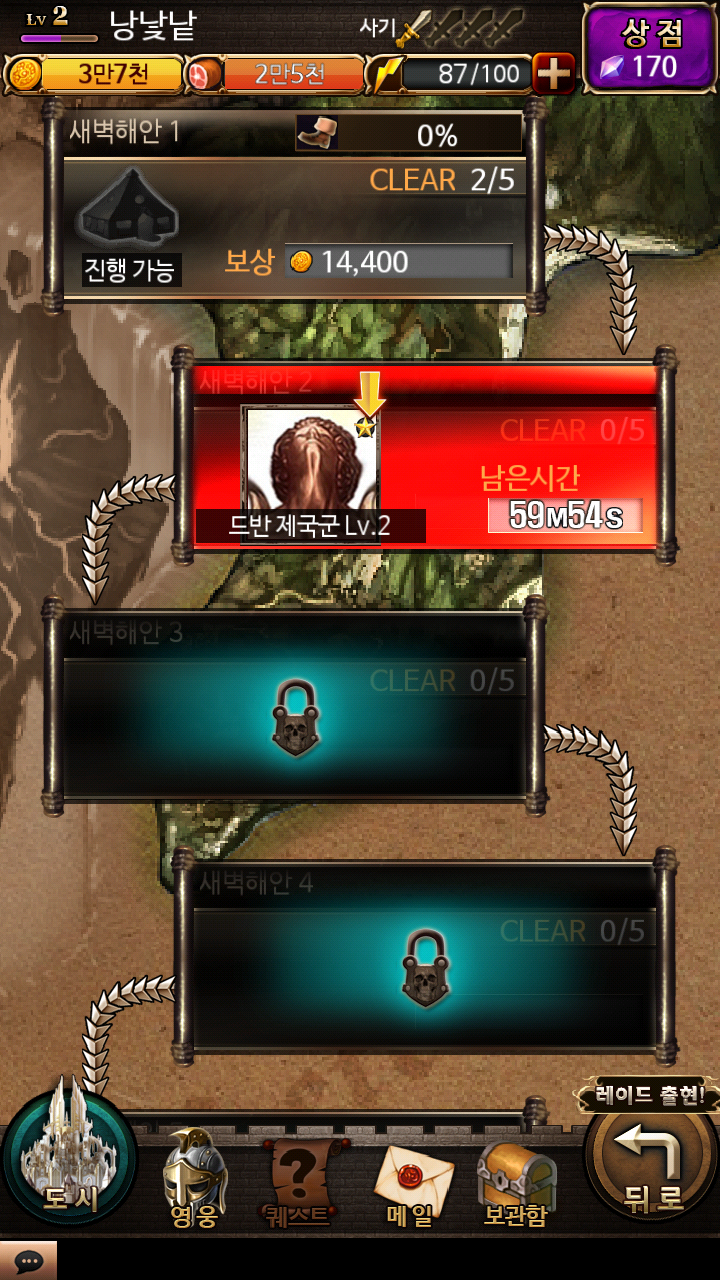This image appears to be a screenshot from an Asian mobile game, possibly written in Chinese or Japanese. The focal point of the image displays four main boxes that seem to represent different game levels or stages, offset slightly to the right or left, connected by metal lines made up of repeating triangles. The top box contains text reading "Clear 2/5," amidst various Chinese characters, and depicts visuals such as a treasure chest and question mark. Below it, there's an avatar alongside other text, while the bottom two boxes are blue and black with locks, suggesting these levels are yet to be unlocked. 

The top right corner of the image features a purple square, and just below it, a black triangle displaying Japanese letters. Across the image, there are other shapes like yellow, orange, red, purple, black, and turquoise triangles containing various stats and text like "Clear 0%," "2 out of 5," and digits such as "14,400" and "5M54S". 

At the bottom, navigation icons featuring designs of a tower, a knight's helmet, a treasure chest, and a letter are visible, likely functioning as menu or navigation buttons within the game. The uppermost section of the image shows character stats, with partially filled bars that probably indicate health, magic, or other gameplay attributes, accompanied by symbols like a sword.